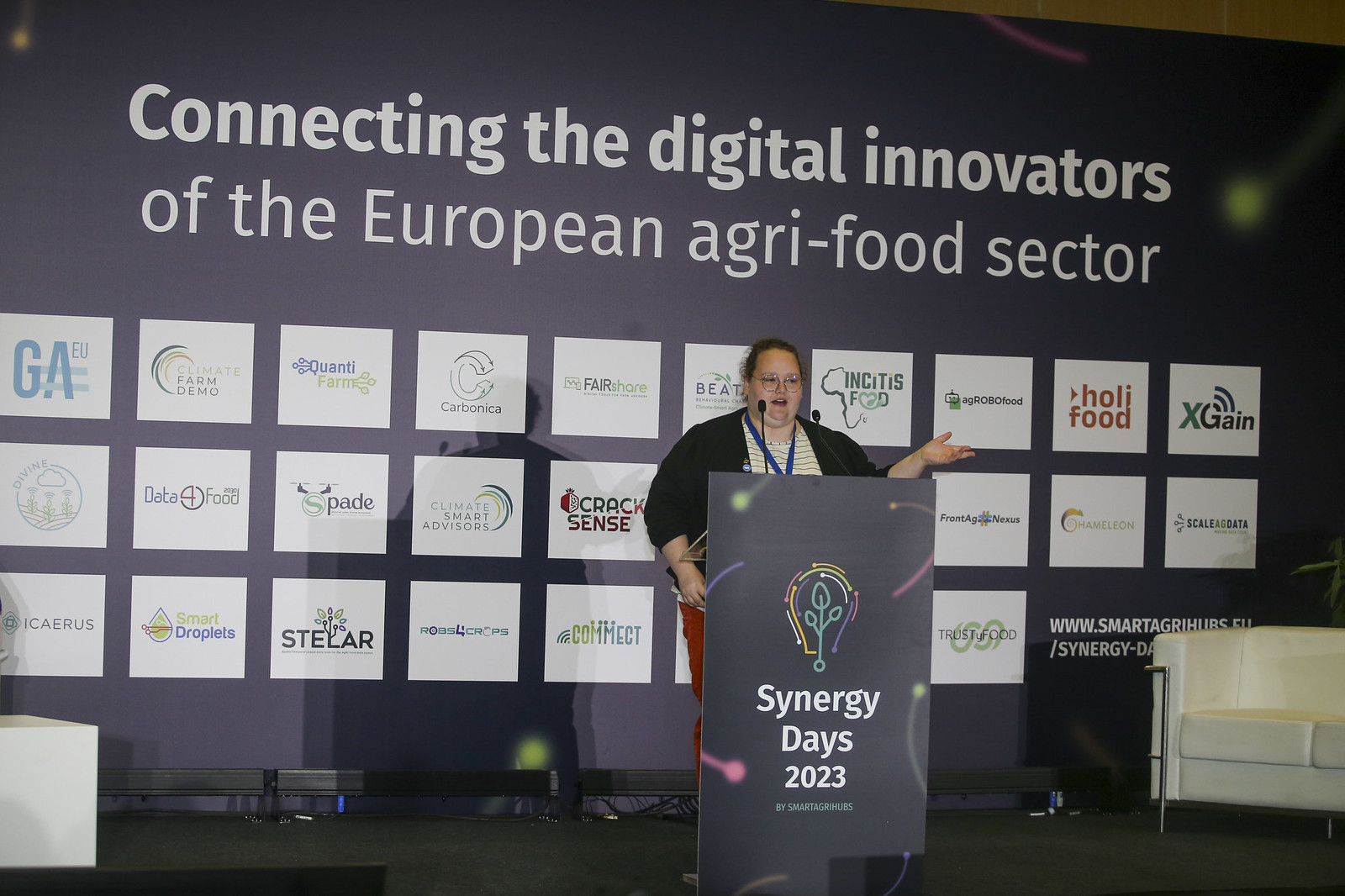In this image, a Caucasian woman is giving a presentation from a podium on a stage. The podium features a rectangular black sign with colorful lines in pink, green, and purple, centered with a lightbulb symbol containing green leaves and the words "Synergy Days 2023." The woman, who is relatively overweight, has brown hair tied back and wears glasses. She is dressed in a black cardigan sweater over a black and white striped shirt, red pants, and a blue lanyard. Behind her is a large navy blue banner with white text at the top that reads, "Connecting the Digital Innovators of the European Agri-Food Sector." The banner lists numerous companies including Holy Food, Stellar, Smart Droplets, Spade, Data Food, QuantiForm, Carbonica, Fair Share, Trust Food, among others.